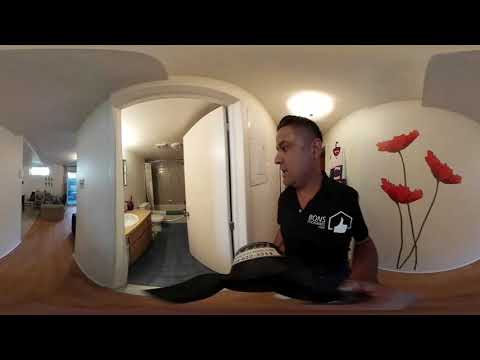In this horizontally aligned rectangular image with thick black borders at the top and bottom, the scene is set inside an apartment or house with white, smooth ceilings and brown wood plank-style flooring. Centrally positioned is a man facing the left, with short black hair that is shaved on the sides. He has brown skin and his mouth is open, possibly caught mid-speech. The man is wearing a short-sleeved black polo shirt featuring a partially visible logo with a thumbs-up design and the word "Bonds" in white lettering, though the exact text is hard to decipher. His bottom half is blurred, but he appears to be holding something. Behind him, adorning the wall, is a painting of three large red poppies that almost reach the ceiling. A white ceiling lamp emits light directly above him. To the left of the man, an open door reveals a bathroom with visible wood cabinets and a sink. Further left, a hallway extends into more open space, likely leading to a living room with a window. The overall setting suggests it is midday and captures a cozy yet detailed snapshot of a home's interior.